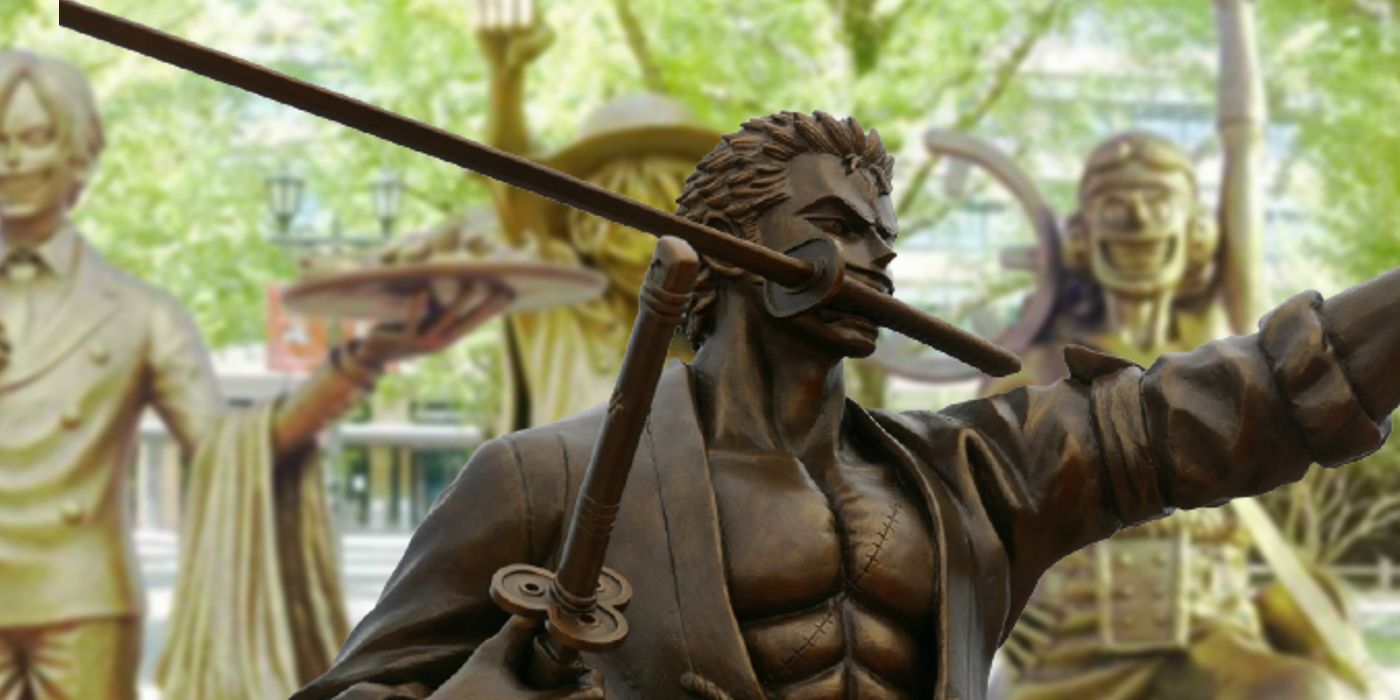In this detailed photograph, the centerpiece is a striking bronze statue of a muscular man with spiky hair. He is depicted from the waist up, his open robe revealing a chiseled chest with a distinctive stitched scar. In his right hand, he holds a sword aloft, its handle pointing skyward. He also clenches another sword in his mouth, adding a dramatic flair to his imposing figure. Surrounding this focal statue are three golden-hued statues, blurred but discernible in the background, set against a leafy backdrop of trees. One of these statues is of a woman with a hat, her fist raised. Another depicts a smiling figure, possibly a waiter or butler, holding a tray aloft. The third, also smiling widely, is similarly clad in a hat and lifting his hand. This outdoor display captures the interplay of metallic sheen and natural surroundings, creating a vivid tableau of artistry and atmosphere.